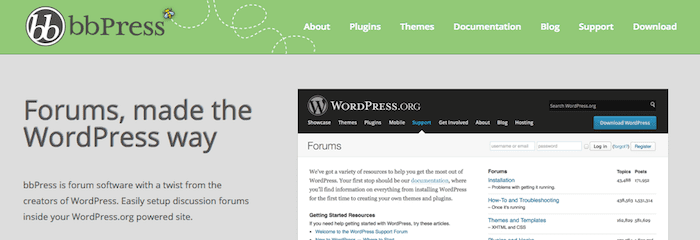The image captures the upper half of a webpage, prominently featuring a bright green header banner at the top. On the left side of the banner, the text "BB Press" is displayed alongside a circular logo containing two interlocking 'B's. The banner includes seven distinct clickable tabs, although their specific labels are not visible.

Beneath the green banner, the background shifts to gray. On the left-hand side of this section, black text reads, "Forums made the WordPress way." To the right, there's a depiction of a webpage, specifically showing a section of the site for wordpress.org. This depicted page has a black banner, with a highlighted "Support" tab in bright blue, while the other tabs remain white. The attention to detail suggests the image is demonstrating how BB Press integrates seamlessly with the WordPress environment for forum management.